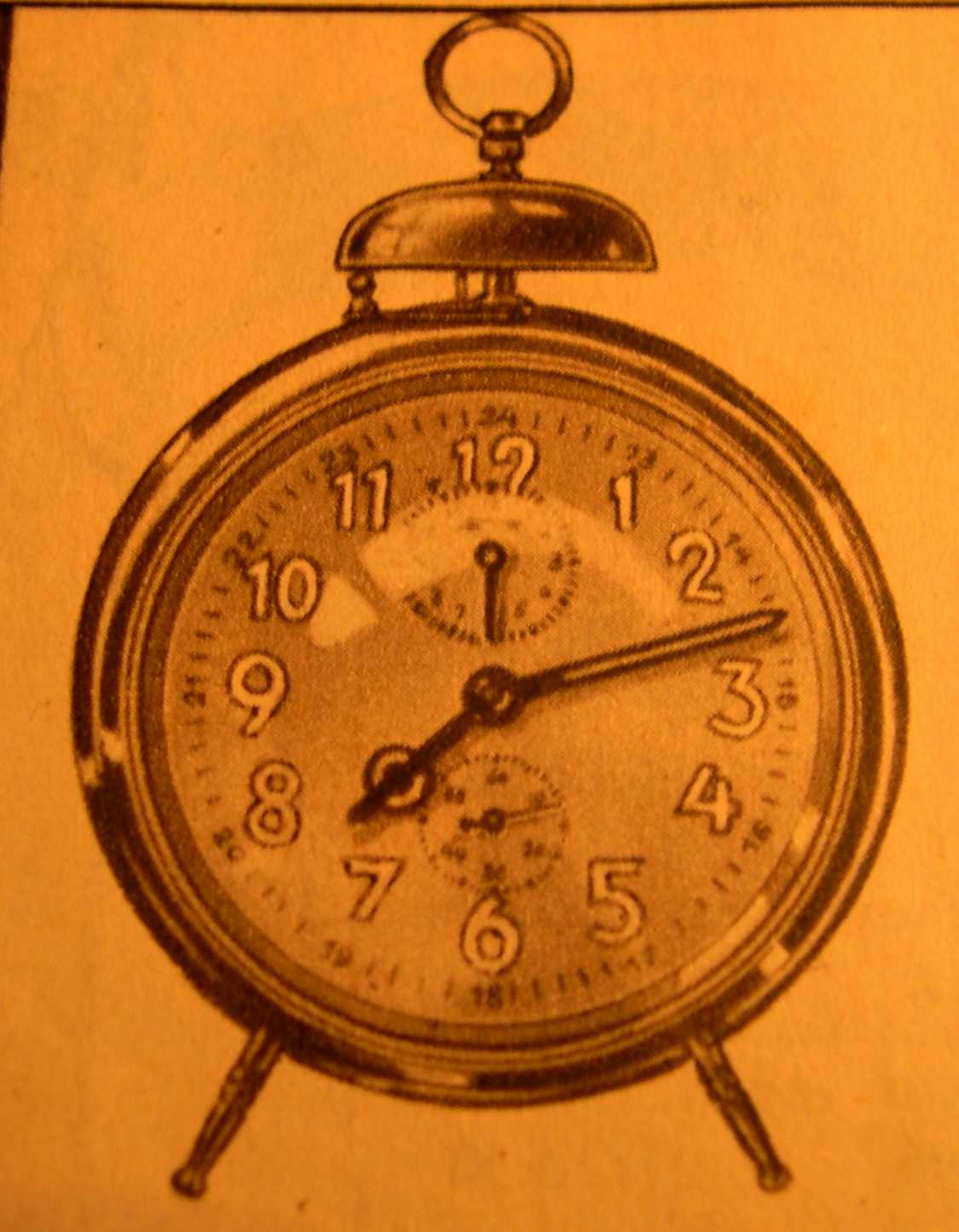This vintage vertical illustration features an old-fashioned alarm clock set against an orange background. The alarm clock, with its classic bell on top, is predominantly brown. It boasts a metallic base where the clock face is mounted. The main clock face displays the time 7:13, with the hour and minute hands in black; notably, the minute hand has an open space within its structure. Below the number 12 and just above the center of the clock hands, there is a separate small dial specifically for the second hand. Additionally, there's another dial that potentially indicates the day, featuring a black needle. The numbers on the clock are outlined in either black or brown and are filled with white, giving them a striking appearance against the brown clock face.